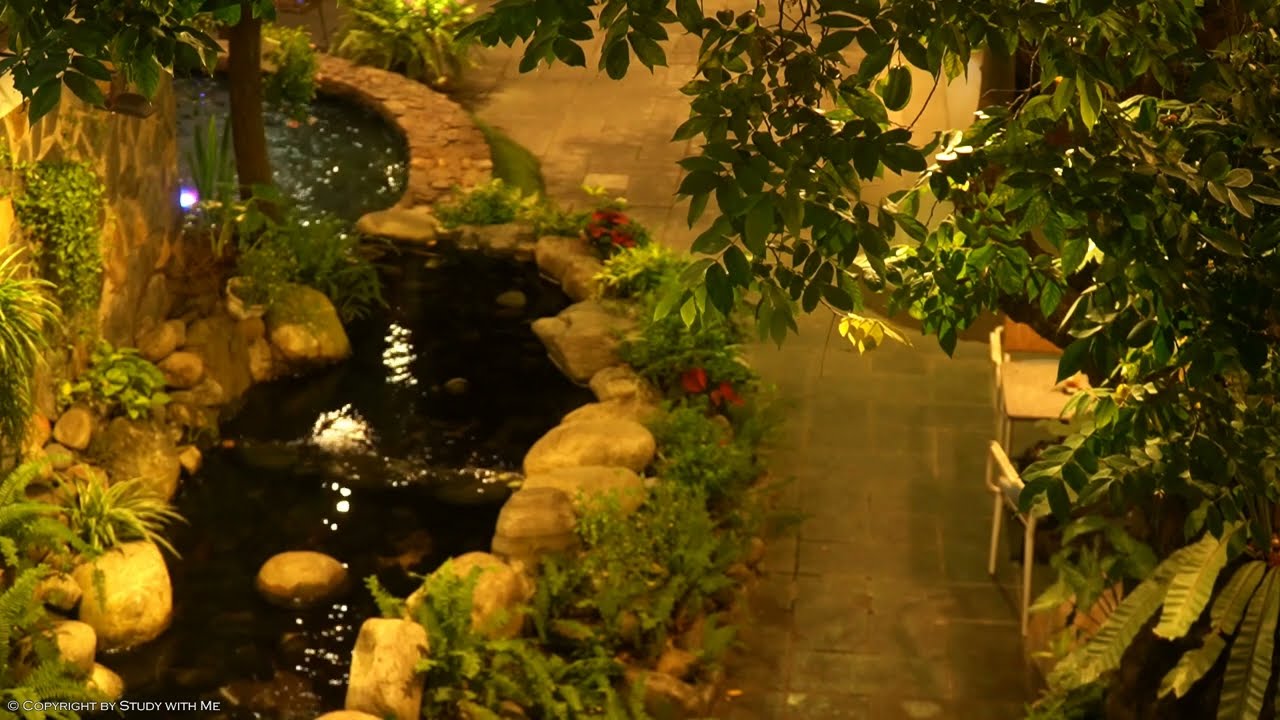The image appears to be taken at night, illuminated with a yellowish hue. It captures a picturesque garden-like area with a man-made stream or pond nestled within a brick and rock enclosure. Lush greenery, including trees with leafy canopies, ferns, and flowers, adorns the scene. A thick tree overhead partially obscures the view. To the right, a stone walkway, appearing wet as if from recent rain, leads through the garden. A chair is visible in the lower right-hand corner, suggesting a place for rest and contemplation. Reflections of light dance on the dark water of the pond-like feature, which has surrounding walls lined with numerous rocks. Overall, the tranquil park or business establishment is artistically framed by nature and masonry under the mellow glow of nighttime illumination.